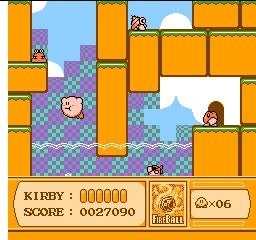The image showcases a screenshot from a classic Kirby video game, likely from the original Nintendo console. In the scene, Kirby, the iconic pink character, is flying on the left side of the frame with his cheeks puffed out, as if he has inhaled air. The environment is rich with platforming elements, featuring numerous yellow platforms scattered throughout the stage. Various enemies populate the screen: a small creature in a shell is situated at the top, a menacing figure with prominent teeth is positioned on the left, and a fish is visible within a body of water beneath Kirby. A distinct brown doorway stands with an enemy character in front of it. The background is adorned with an assortment of geometric shapes, comprising blue blocks and yellow-green squares set against purple blocks. The upper portion of the image displays a vibrant blue sky with fluffy white clouds.

The game's user interface (UI) is visible at the bottom of the screen. It includes a section labeled "Kirby" with notches beside it, a score displayed as "0027090," an icon labeled "Fireball," and a small image of Kirby next to the notation "x 06."